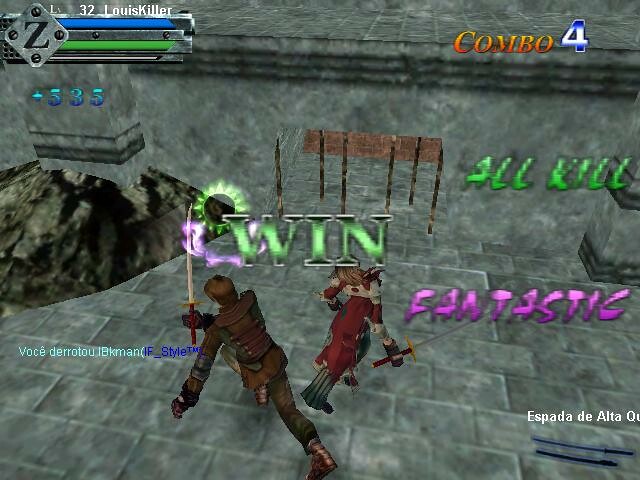This detailed screenshot from a video game features a central battle scene on a floor made up of gray and light gray tiles. The area has blocky, castle-like square pillars along the sides and another level of gray floor tiles in the background. 

In the center, two characters are shown from the back. The character on the left, identified as Louie Killer (Level 32), is a male with brown hair, wearing a brown jacket, and holding a sword in his right hand. His left arm is extended to his side, and his right leg is stretched out behind him, suggesting he is running or lunging to the left. The character on the right is a female with light brown hair, wearing a long reddish skirt, bent elbow, and holding a sword in her right hand, facing toward the right.

The interface highlights various in-game statistics and notifications: 
- The top left corner displays the player's name, "Louie Killer (Level 32)," accompanied by a metallic plate showing a blue bar with a green bar underneath, and a score of "+585" in blue text.
- The top right corner shows "Combo" in orange text with the number "4" beside it in blue.
- In the upper center, the word "WIN" is prominently displayed in green.
- The upper right corner also reads "All Killed," and the bottom right corner says "Fantastic."
- The bottom left corner mentions a role that could be "Voice Director" or similar.
- The bottom right corner identifies "Espada Delta."

The overall scene is predominantly gray, with the victorious male character in pants having seemingly won the game.